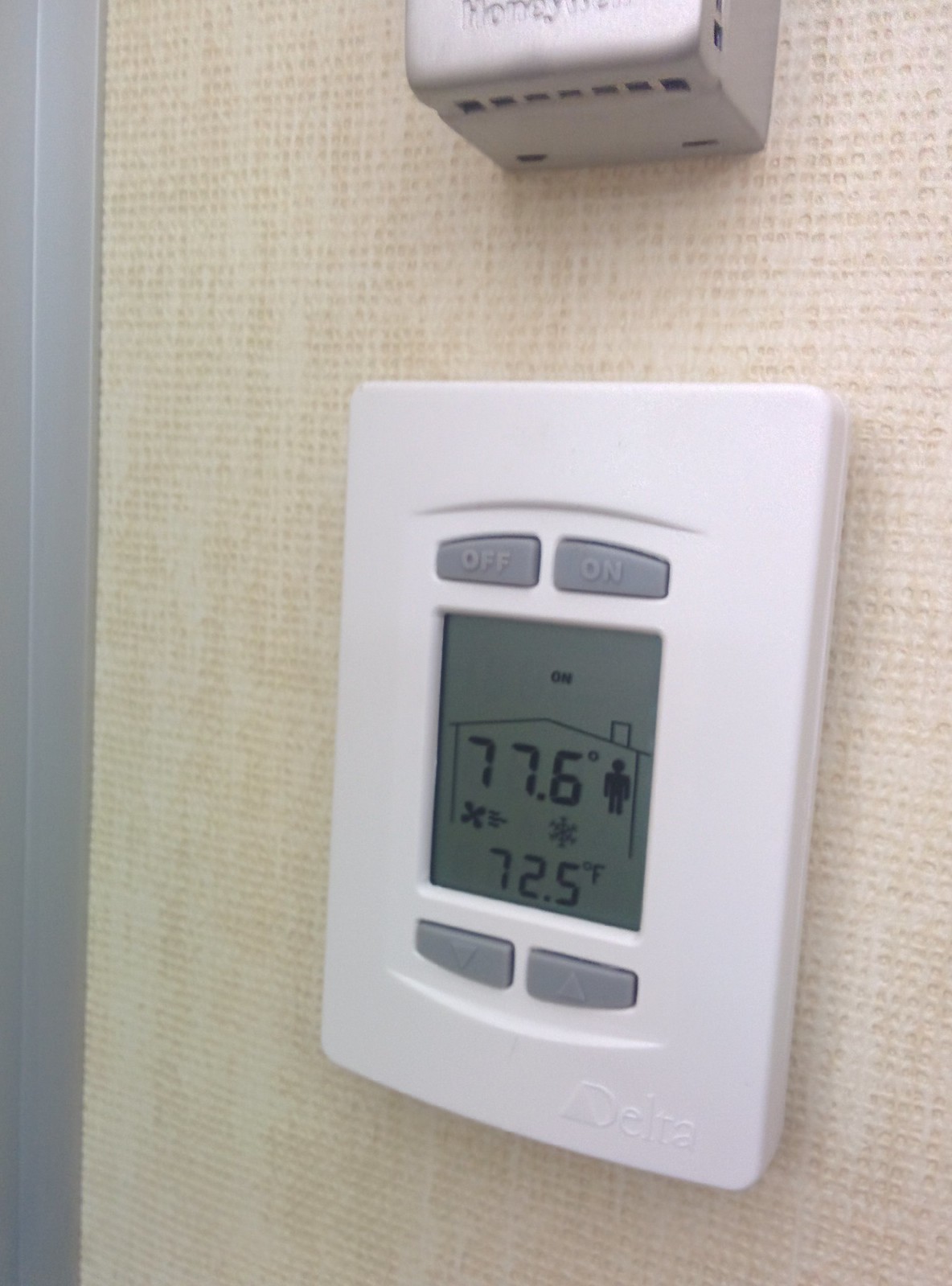In this detailed colored photograph, a rectangular white thermostat is prominently displayed against a wall made of light brown woven material. The thermostat is mounted vertically and features two buttons at the top: a gray "Off" button and an "On" button. Below these are two more buttons for adjusting the temperature, labeled with downward and upward arrows.

The device's display screen has a light grayish-green hue, showing a current temperature reading of 77.6 degrees Fahrenheit. Above the temperature, there is a small icon depicting a person, while to the right side of the screen are icons of a fan and a snowflake respectively. Below this information, the set temperature is shown as 72.5 degrees Fahrenheit. At the very top of the screen, the status "On" is clearly visible.

Branding is minimal but noticeable, with "Delta" inscribed at the bottom right corner of the device. A few inches above the thermostat, also on the wall, there is a square protrusion of an unidentified object or control panel, partially cut off from the frame, adding an element of curiosity to the overall scene.